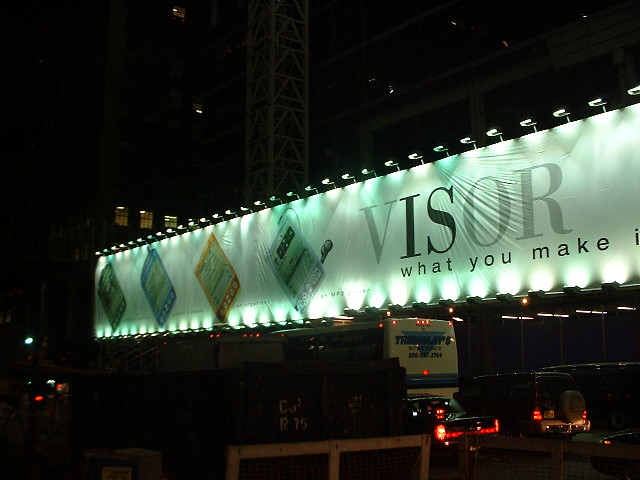This color photograph, captured at nighttime, presents a bustling urban scene centered around a massive, horizontally-stretching billboard. Positioned prominently across the center of the image, the billboard is vividly illuminated by lights at both its top and bottom edges. Its backdrop is a dark, night sky, suggesting a densely built metropolis with a hint of calm.

Underneath the billboard, a large yellow bus is visible, dwarfed by the towering advertisement above. Several cars, their headlights piercing the night, add life to the scene, lined up directly beneath the billboard. A towering skyscraper or tall structure looms in the background, providing a stark contrast to the brightly lit sign.

The billboard itself is a striking green shade, drawing immediate attention. On the left side, four square objects, slightly tilted to the left, punctuate the design. In bold gray and black text across the sign are the words: "visor, what you make it." The right edge of the billboard crops the 'T' in 'it', giving an impression of continuity beyond the frame. A subtle detail, the fabric of the billboard, is slightly pulled over the 'S' and 'R', adding a touch of realism to the otherwise pristine surface.

The overall effect is a dynamic depiction of an urban nightlife scene, characterized by its blend of glowing advertisements, vehicular movement, and towering structures.